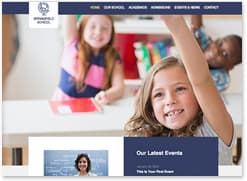This image is a low-quality screenshot of a website's homepage, featuring a navy blue top menu bar. The menu text is unreadable, but the background color is clearly navy blue. On the left-hand side of the menu, there is an illegible company name written within a white triangle. The main focus of the image is three children, suggesting that the website could be for a school, an online educational platform, or a tutoring service.

In the foreground, to the lower right, is a white girl with brown hair and a big smile, appearing to be around 10 years old. She has a black background and is closest to the camera. Behind her and slightly out of focus is a boy with medium to dark skin, possibly also around 10 years old, wearing what seems to be a turquoise and navy blue plaid shirt. To the left of the boy is another girl with reddish-brown hair who is smiling as well. She is wearing a shirt with large horizontal stripes in blue and pink. All three children are raising their hands as if in a classroom setting, adding to the educational theme of the website.